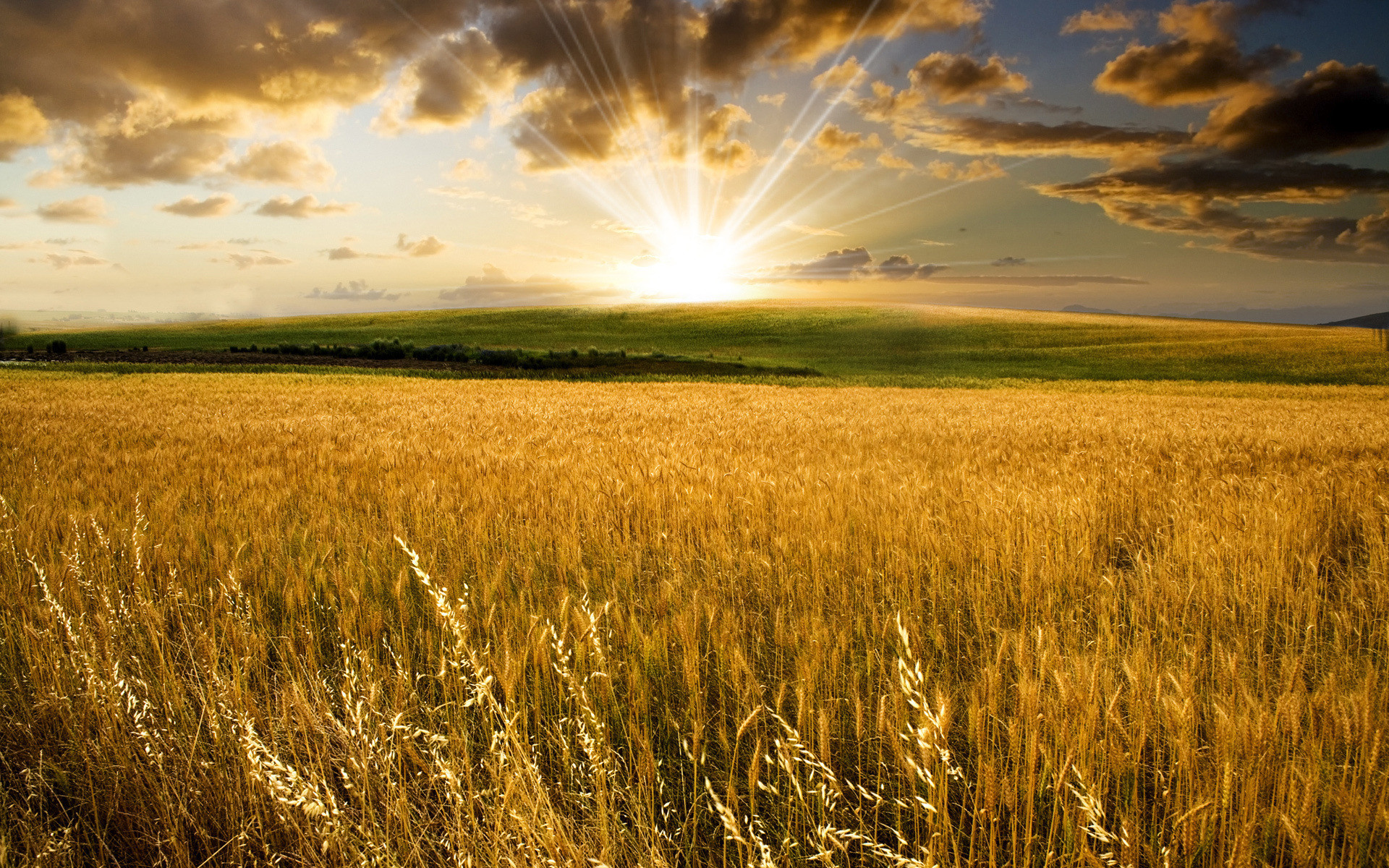The image captures a serene scene of a sunrise over a vast wheat field. The photograph is horizontally aligned, with a beautiful sky dominating the upper portion. The sky transitions from a light blue on the left to a darker blue on the right, interspersed with puffy white and gray clouds. At the center top of the image, a circular yellow sun emits radiant rays in various directions, casting a warm glow over the landscape. Below the sun, a green hill with smooth grass and scattered shrubs extends across the scene. In the foreground, tall, golden wheat plants with seed heads sway gently, adding to the tranquility. A stone fence divides the fields, adding texture and depth to the composition. The image captures the beauty and calm of a sunrise over a pastoral landscape.